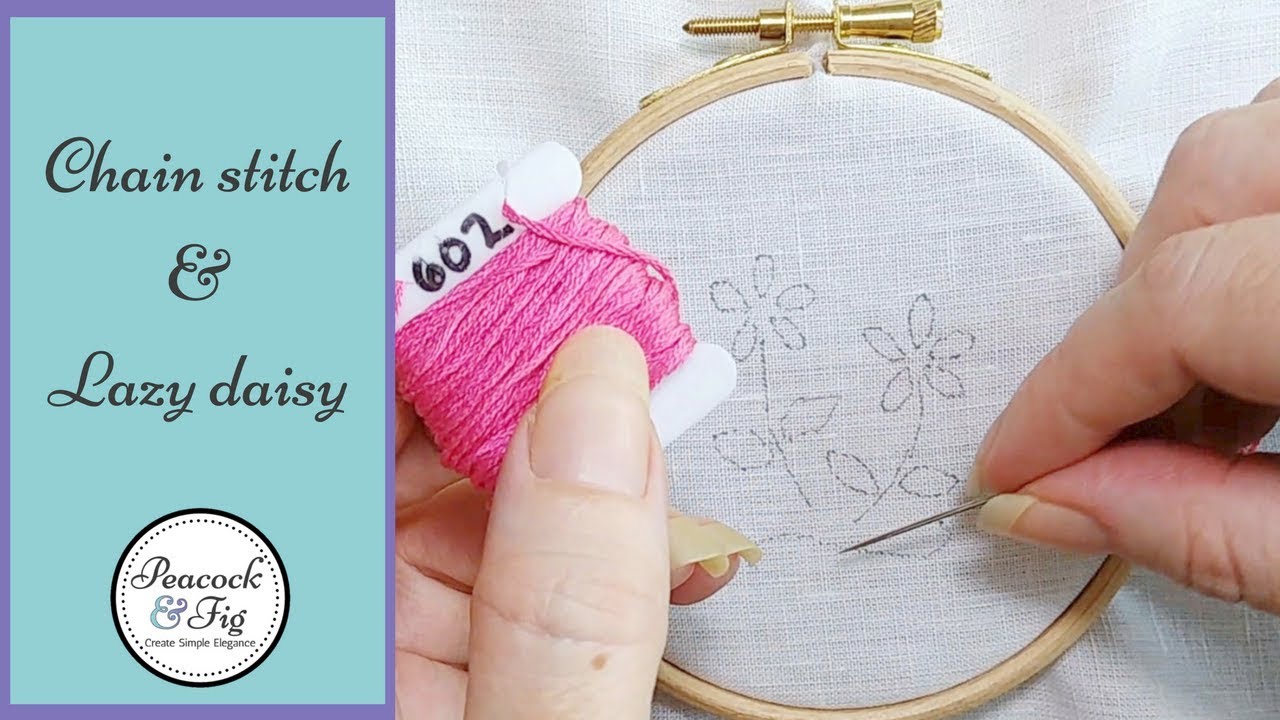In this detailed image, we observe a person intricately engaged in needlepoint embroidery. The fabric is securely fastened in a wooden embroidery hoop, and they are stitching a series of flowers using a chain stitch and Lazy Daisy techniques. The thread in use is a vibrant pink, specifically noted as color number 602, which is wrapped around a piece of cardboard. The person has long fingernails and is holding the thread with their left hand while their right hand maneuvers the needle. A turquoise-colored rectangular sidebar on the left side of the image features a circular logo that reads "Peacock and Fig, Create Simple Elegance" in a black cursive font, with additional text indicating the stitching techniques "Chain Stitch" and "Lazy Daisy" in the same stylish script.